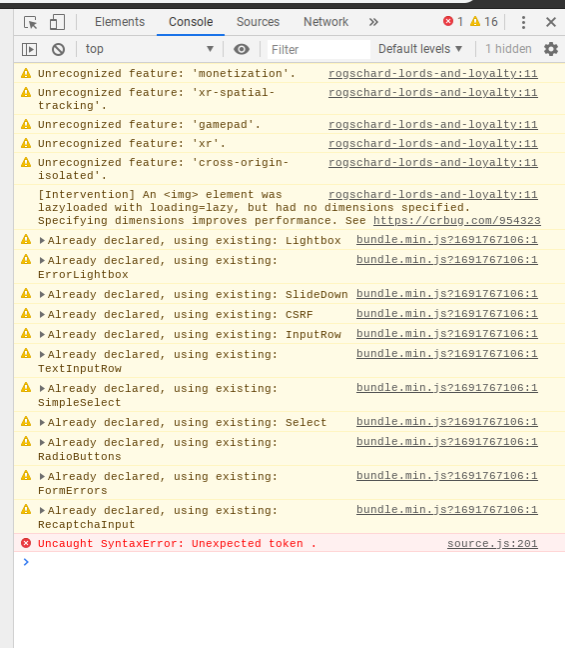The image is a screenshot of a browser's developer tools console set against a light gray background. In the upper left corner, there are several menu elements arranged from left to right: "Console" (underlined in blue, indicating it's the active tab), "Sources," and "Network." Following these are a notification indicator displaying the number "1" and a yellow triangle with the number "16."

Below these menu elements, the word "Top" is visible, under which there is a filter input box and a drop-down menu labeled "Default levels." The term "1 hidden" is displayed, suggesting certain console messages are not visible. To the right of these options, there is a settings icon.

The main section of the console is filled with numerous lines of script. Each line begins with a yellow triangle, signifying a warning or error. Following the script on each line, there is a clickable blue underlined link. For example, the first line contains a link labeled "ROGS Chard Lords and Loyalty 11."

This detailed display within the console suggests the user is debugging a web page and is being alerted of multiple warnings or errors within the script.